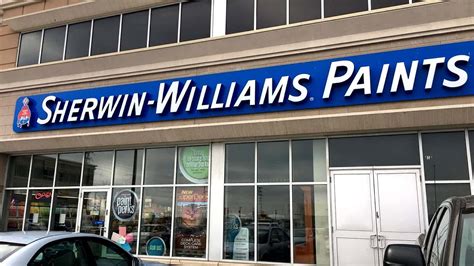This vibrant, horizontally-oriented color photograph could easily serve as an advertisement for a website. It captures a light brown brick building with a row of dark gray windows on the upper portion, framed by white outlines. Centrally placed slightly above the middle of the image, a prominent blue banner with raised white 3D lettering reads "Sherwin-Williams Paints," accompanied by a raised logo to the left of the text. The storefront beneath this banner features large glass windows and a white door, displaying several signs within the window reflections. In the lower left corner of the image, a silver car is parked, while the lower right quadrant reveals a white set of double doors and the partial view of a gray car with a black side mirror. Sunlight bathes the entire scene, causing the windows to reflect the surrounding parking lot in an array of rainbow and pastel colors.